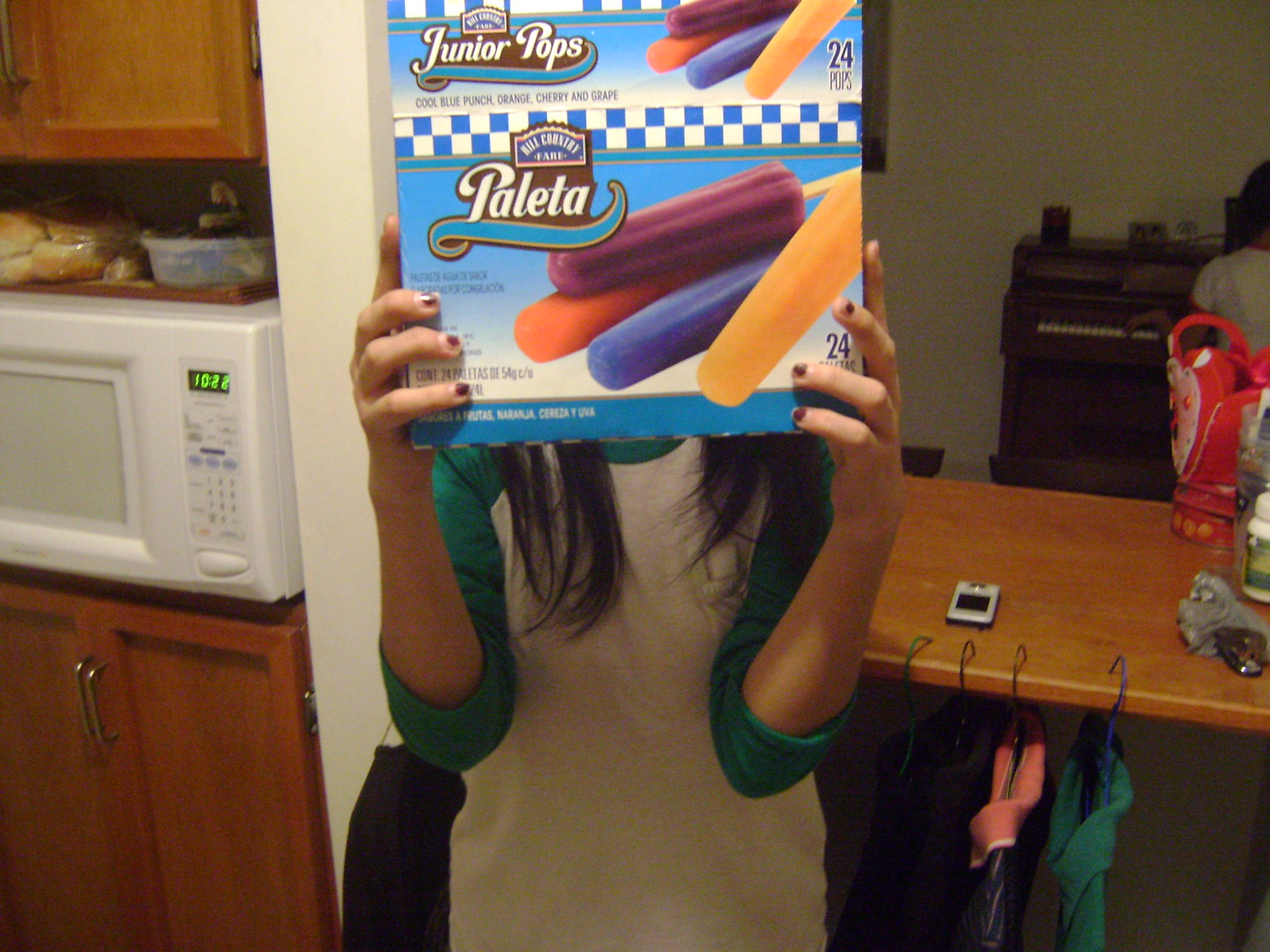In this detailed kitchen scene, a young woman is holding a box of Hill Country Fair Paleta popsicles above her head, obscuring her face. The box features colorful popsicles in purple, orange, blue, and yellow, designed with a blue and white checkerboard pattern and white shading. The woman has long dark brown hair and chipped fingernail polish, wearing a green long-sleeve shirt with the sleeves rolled up to the elbows and a white shirt underneath. Behind her, a typical kitchen setup is visible, including a white microwave nestled between brown wooden cabinets. To the right, a brown wooden table holds a few different appliances or baskets and has clothes hanging on hangers. In the background, a brown wooden piano with white ivory keys is against a tan wall, contributing to the homely, cluttered atmosphere.